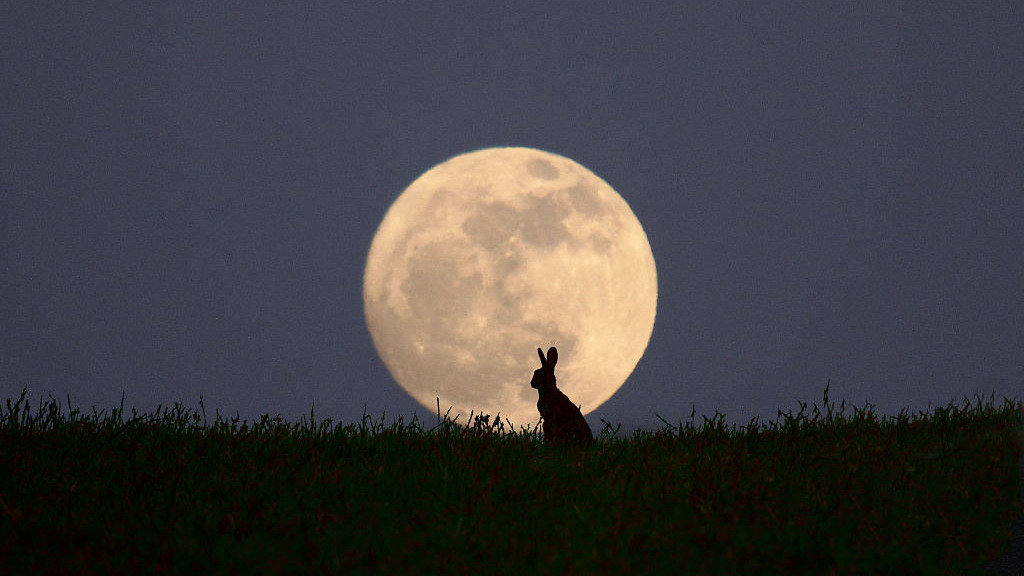In the serene nighttime image, a dark blue sky stretches across the backdrop, with the full moon appearing to rest gently on the horizon, casting a soft glow. Shades of gray ripple through the luminous moon, which dominates the upper center of the image. Below, dark grass extends upward, its color indistinguishable in the dim light, adding texture to the scene. The focal point, framed perfectly by the moon's light, is the silhouette of a rabbit, possibly a jackrabbit. Sitting upright with prominent ears, the rabbit's outline is clearly visible, creating a striking contrast against the glowing moon, and evoking a sense of tranquil solitude in the night.